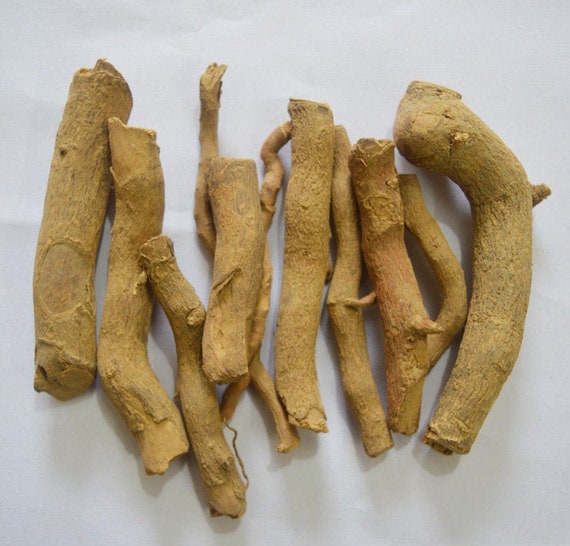The image depicts ten knobbly, branch-like objects of varying thicknesses and shapes, approximately 6 to 7 inches long. These objects resemble unshaved ginger or tree branches, arranged side-by-side with some slight overlapping on a white background that could be paper. Their colors range from dusty yellow to brownish-yellow, akin to turmeric powder. Each piece exhibits unique imperfections such as curves, dense areas, or additional small offshoots, giving them a distinctive but cohesive appearance.